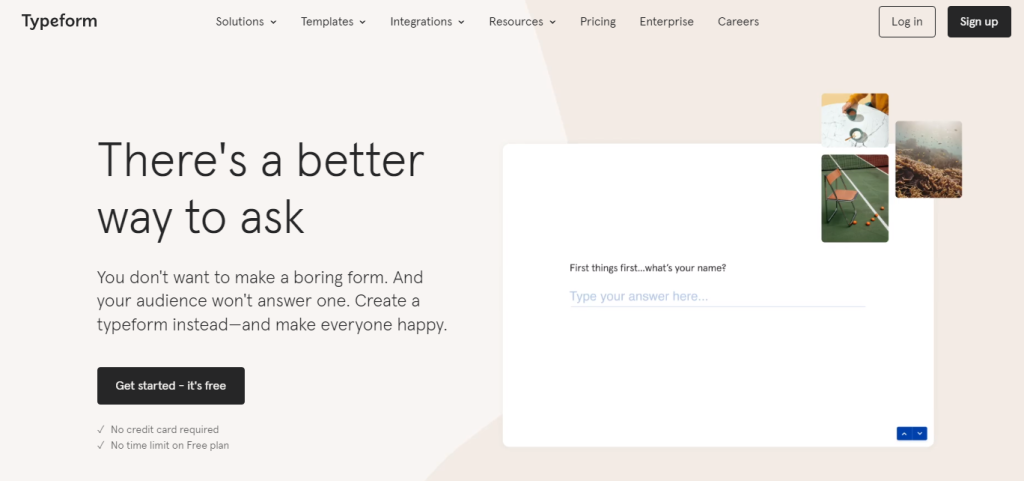This image is a promotional screenshot from Typeform, featuring a sleek layout against a muted grayish-tannish background. At the top of the interface, there are navigation options for "Solutions," "Templates," "Integrations," "Resources," "Pricing," "Enterprise," and "Careers," with the first four options having drop-down menus. A "Login" button and a black "Signup" button are prominently displayed for user access. 

The central body of the page boasts the slogan: "There’s a better way to ask," underscoring Typeform's user-friendly alternatives to mundane forms. The accompanying text emphasizes the advantages: "You don’t want to make a boring form and your audience won’t answer one. Create a Typeform instead and make everyone happy." 

A call-to-action button beneath this text urges users to "Get started. It's free," also in black, with highlights noting "No credit card required" and "No time limit on the free plan." 

Adjacent to this, a white pop-up box introduces a sample form, posed with the initial question: "First things first, what's your name?" Below the query, a prompt in blue reads "type your name here," with a text input field provided. This interface also features three small photographic thumbnails: one depicting a chair, another showing plants, and the third showcasing a landscape, contributing to the aesthetic appeal of the form.

In the lower right corner of the pop-up box, a blue button with up and down arrows allows for easy navigation through form fields. This intuitive design highlights Typeform's mission to simplify form creation and enhance user engagement.